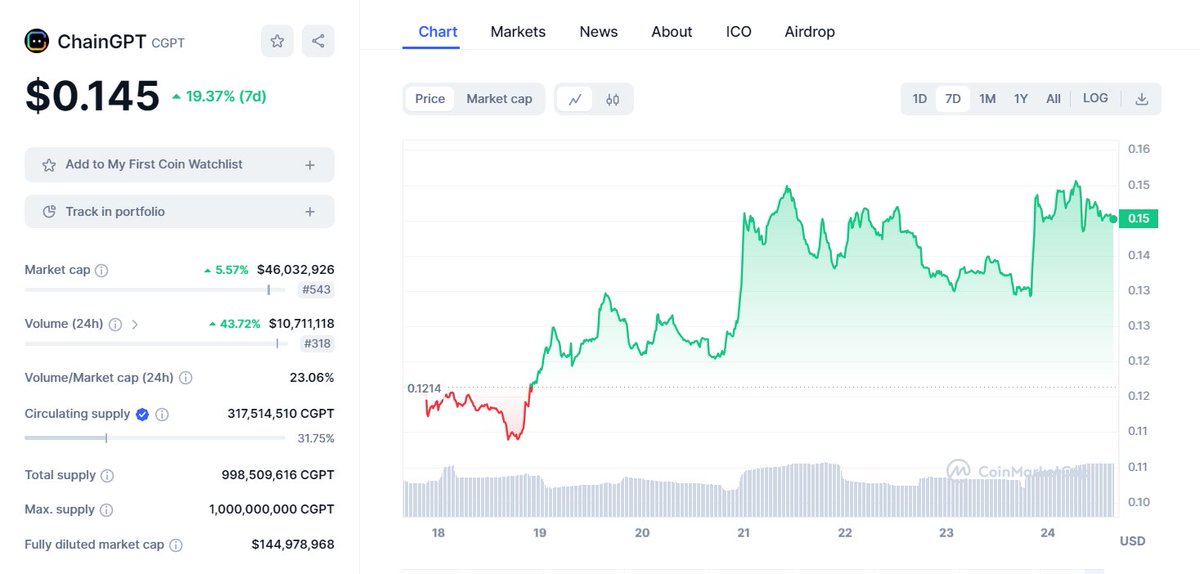Screenshot of a Bitcoin/Cryptocurrency Platform - ChainGPT

This detailed screenshot displays the user interface of a cryptocurrency platform specializing in ChainGPT. Dominating the top left corner, the platform's name "ChainGPT" is prominently displayed alongside its logo. The logo features a black background with a rainbow square border on the inside and two white dots.

Beneath this, the current price of ChainGPT is listed as $0.145 with a small blue upward arrow indicating a 19.37% increase over the last 7 days, denoted by "(7D)".

The top menu bar features navigational options such as Chart, Markets, News, About, ICO, and Airdrop, allowing users to easily explore different sections of the platform.

The central focus of the page is a detailed graph tracking the coin's performance over the past seven days. The graph shows the coin initially in the red but climbing closer to the current day, with a high point of $0.15 and a low point of $0.1214.

Down the left sidebar, the page provides crucial financial metrics such as Market Cap Volume, 24-Hour Market Cap, Circulating Supply, Total Supply, Max Supply, and Fully Diluted Market Cap. The bulk of the text is in black, while hyperlinks are in a distinct blue. Sage green is also used prominently on the graph and in various financial indicators, adding vibrancy and visual clarity.

This comprehensive view offers a snapshot of ChainGPT's recent performance and essential data for users and investors.